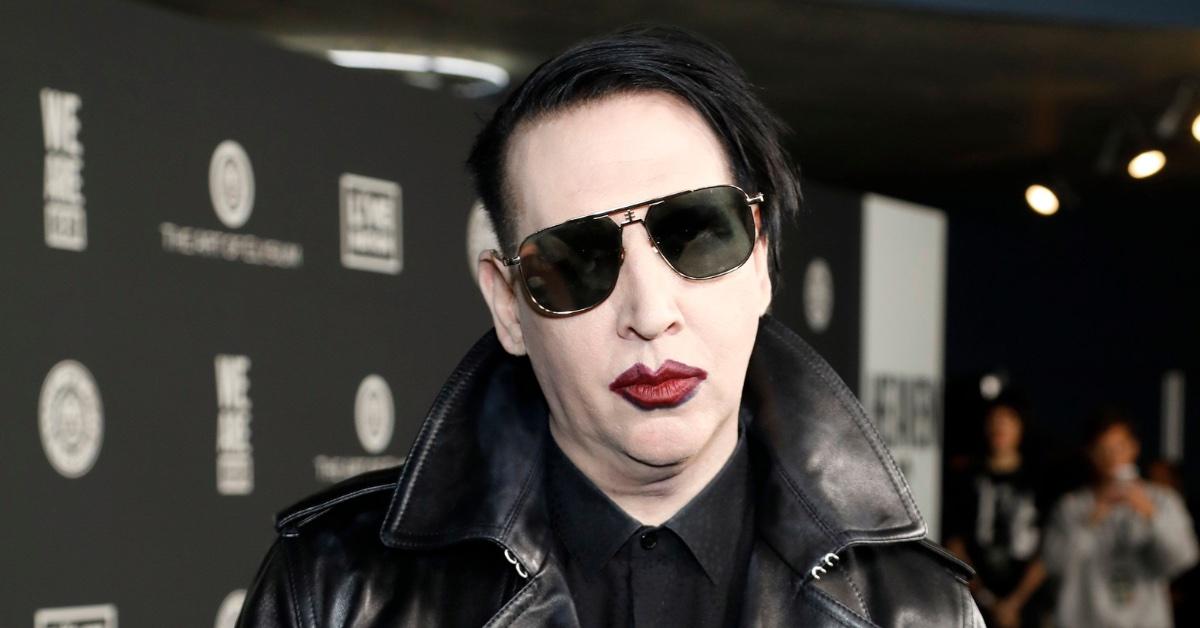In this image, the musician-artist Marilyn Manson stands at the center, exuding his iconic gothic look. His dark black hair is styled with a swoop to one side, contrasting sharply against his almost ghostly pale skin. He wears his trademark black aviator sunglasses, which slightly tilt, and draws attention to his striking red lipstick. His outfit consists of a black button-down shirt with a pulled-up collar, layered under a black leather jacket. The background is indicative of a red carpet event or similar high-profile occasion, featuring a black wall adorned with various white logos and sponsor markings, though the exact details of these logos are indistinct. Blurred figures in the distance are seen attempting to capture pictures, emphasizing the public interest in his appearance. Manson's expression suggests a blend of nonchalance and detachment as he faces the camera directly.